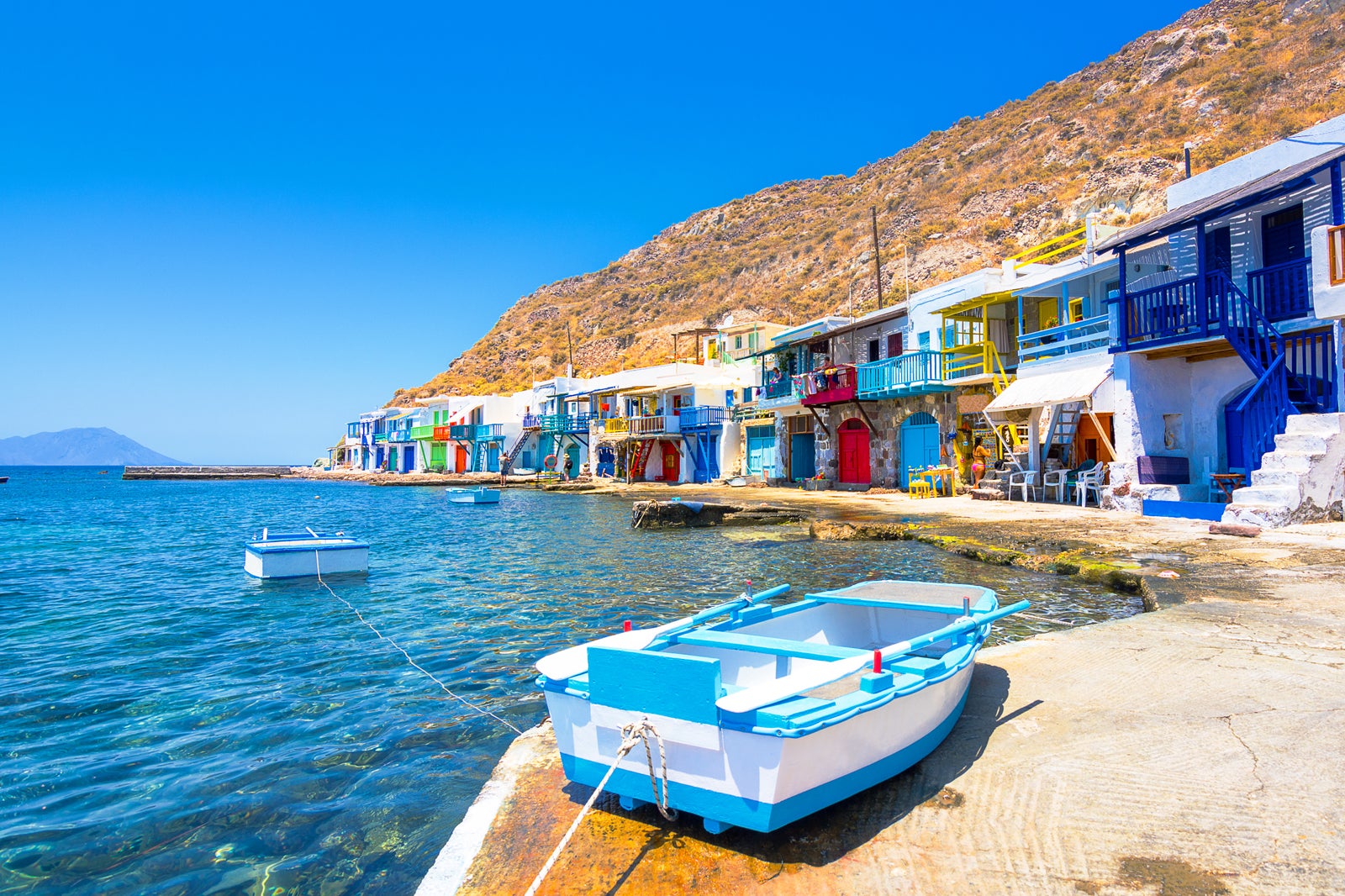This color photograph captures a vibrant and picturesque seaside village nestled at the base of a steep, rocky cliff. A row of charming two-story homes, painted primarily white or beige, stands out with their colorful balconies, porches, and doors—sporting hues like navy blue, yellow, red, orange, and lime green. These houses sit right at the edge of the ocean, with only a few feet of ground separating them from the clear, inviting greenish-blue waters. In the foreground, on a concrete walkway, rests a small white and light blue rowboat, tied with a rope to a floating platform just off the shore. The backdrop features a lush, light-colored cliff, and to the left of the image, the serene blue ocean stretches out, with a distant blue mountain visible under a perfectly blue sky. The scene evokes the charm of a quaint Greek seaside village, complete with a peaceful and inviting atmosphere.